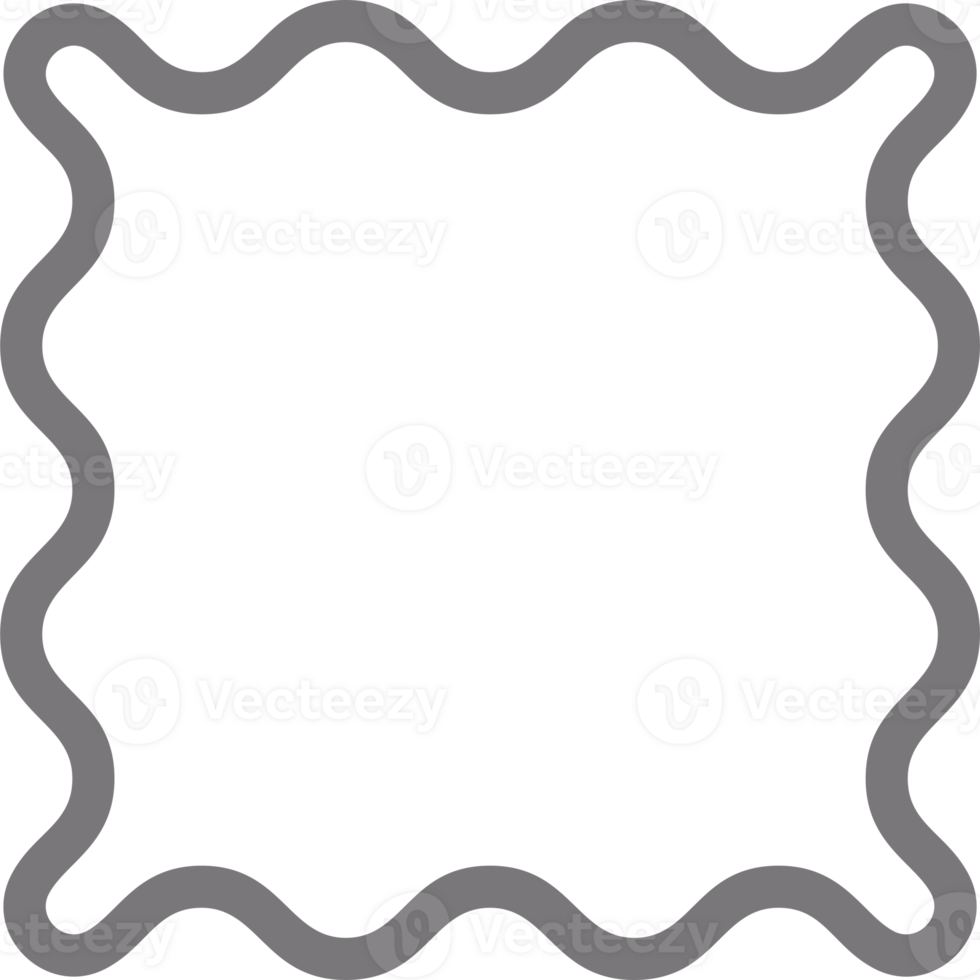The image portrays a detailed, abstract, color drawing of a border frame with an undulating, squiggly line pattern. The border, which is dark brown in color, meanders fluidly with curves resembling the letter 'S' or 'U-turns,' creating a continuous, flowing perimeter with three inward and two outward bumps on each edge, seamlessly connecting at the corners. This intricate design, reminiscent of wrought iron work, surrounds an entirely white background. Overlaid on this border pattern is a repetitive watermark of the text "V-T-Z" or "V-E-E-T-E-E-Z-Y," along with a small stamp resembling a thread in an S-curve. This watermark appears dozens of times, with at least 13 to 14 instances visible, blending subtly into the design and adding a layer of texture to the image.